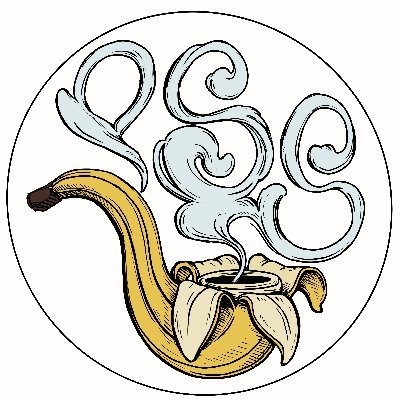This image is a digital animation with a central circular design, outlined by a black ring set on a white background. Within the circle, the main feature is a surreal, abstract depiction of a pipe that has been crafted from a banana. The banana pipe, colored in a washed-out yellow with white peeling around the bowl, mimics the appearance of an actual banana with detailed lines accentuating the fruit-like texture. The bowl of the pipe, located at the top where the banana would be peeled open, is black, and the mouthpiece appears to be the stem of the banana. 

From the pipe, silverish gray, light blue smoke emerges in delicate, wispy curlicues, rising and filling the top half of the circle. The smoke appears to form some abstract, misty letters, possibly "O-S-S." The whole composition is artistic, giving off a vibe that might be associated with a logo for a head shop or a weed company, due to its unique and imaginative design merging everyday fruit with the concept of a smoke pipe.